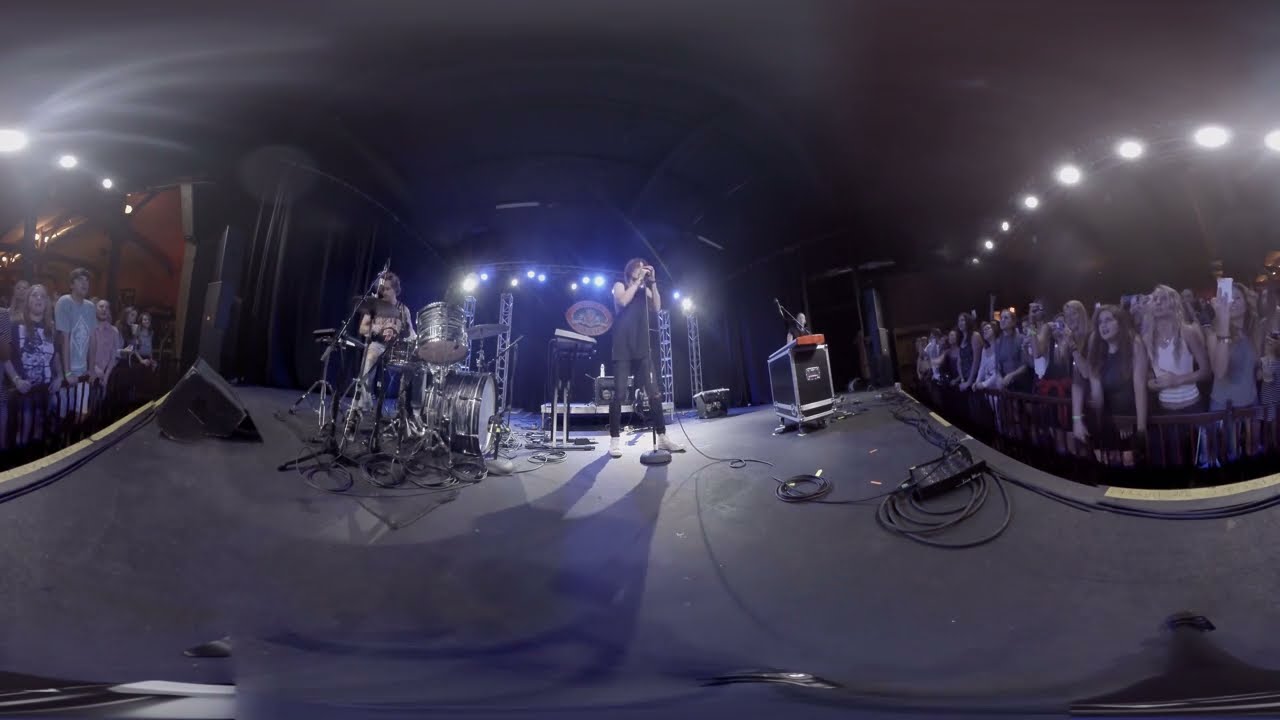In this striking and immersive concert photo, the scene appears to be indoors and was captured using a wide-angle lens, creating a distinctive 180-degree curvature that warps both the stage and the crowded audience on either side. The black stage features a silver drum set and a drummer, whose attire remains indistinct. Another individual stands center stage, clad in a black tank top, black pants, and white shoes, surrounded by a maze of wires and amplifiers. Overhead, a multitude of artificial lights illuminates the scene, reflecting off the black ceiling and casting a dynamic glow on the performers and spectators alike. The audience, visible on both sides and extending far back, stands engrossed in the live music experience, creating an electric atmosphere enhanced by the unconventional, VR-like lens distortion.